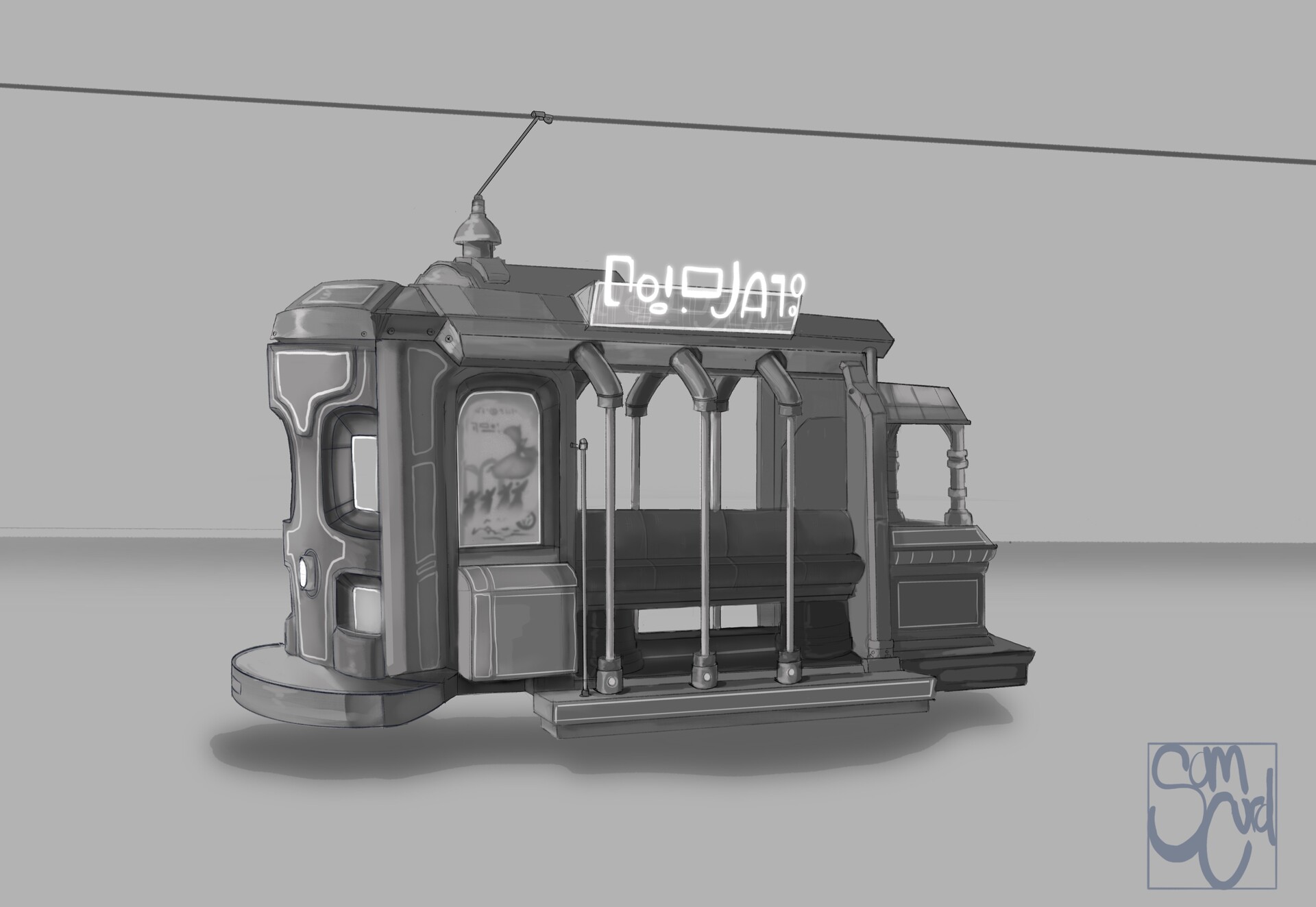This is a detailed, black and white illustration set against a flat gray background. It depicts a futuristic, modernistic trolley or cable car with a distinct hovering quality, as it has no visible wheels or tracks. The vehicle is suspended from a single horizontal cable running across the top of the image, connected by a smaller vertical cable to a bell-shaped dome on top of the car. This conveys its likely function as a transit device hovering above the ground, emphasized further by the shadow beneath it.

The trolley features three vertical poles and seating areas, suggesting that passengers can enter and sit comfortably. There is an open-air section on the left, alongside what appears to be either a picture or advertisement. On the rounded left side of the vehicle, windows provide a view for passengers to gaze outside, while the right side has an almost architectural, house-like exterior.

Above the trolley, there is mysterious, futuristic text in white letters, "D-O-L-O-J-A-1." In the bottom right corner of the illustration, enclosed in a square, the artist's name, "Sam Kurd," can be seen, with the initials "S" and "C" prominently featured. Overall, the piece presents a blend of futuristic and steampunk-like elements, creating a captivating vision of what modern urban transit could look like.